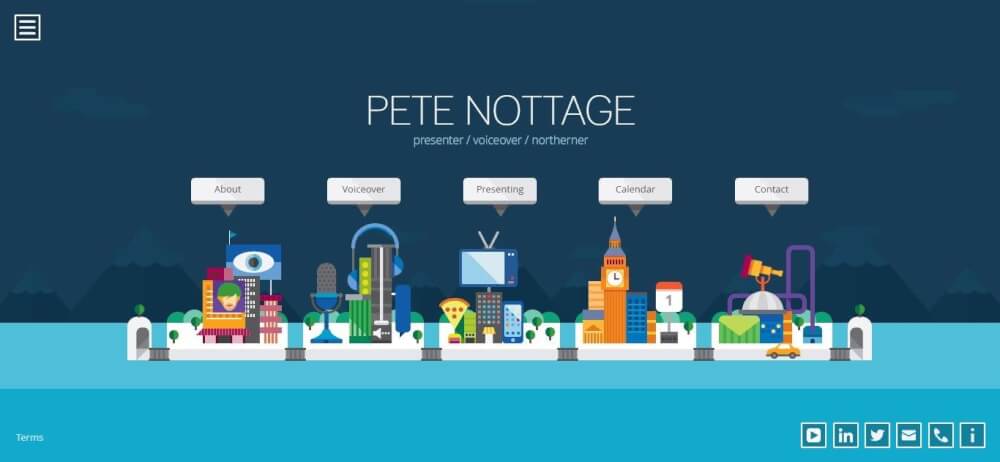The image depicts the website of Pete Nottage, prominently showcasing his name in white capital letters at the center, with "presenter / voiceover / northerner" written underneath in smaller, light blue text. The website features a dark blue background designed to resemble a night sky, complete with illustrated clouds, mountains with snowy peaks, and silhouettes of tree tops. At the bottom, an abstract representation of water is crafted with two shades of turquoise.

Below Pete's name and occupation, there is a navigation bar with five buttons, each featuring a clickable icon that corresponds to different sections of the site, set against illustrated backgrounds:

1. **About**: A colorful icon depicting a man with green hair, a building, and a flag with an eye symbol, positioned above a platform with shrubbery.
2. **Voiceover**: Depicts a microphone and headphones alongside a confusing detail that resembles a wine glass with a spongy element, suggesting a creative interpretation of audio equipment, with surrounding buildings.
3. **Presenting**: Features a TV with rabbit-ear antennas, a slice of pizza, a smartphone, and a building, surrounded by shrubs.
4. **Calendar**: Shows a clock tower, a calendar icon labeled with the number "1", and various buildings against a shrubbery backdrop.
5. **Contact**: Includes a colorful array of icons such as a paintbrush on a metal globe, a house with an arch, and multiple envelopes in green, blue, and orange.

In the lower right corner, social media icons for YouTube, LinkedIn, Twitter, email, phone, and information are displayed within blue squares, utilizing white icons. The overall design is visually engaging and packed with unique, illustrative details that reflect Pete Nottage's professional profile and personality.